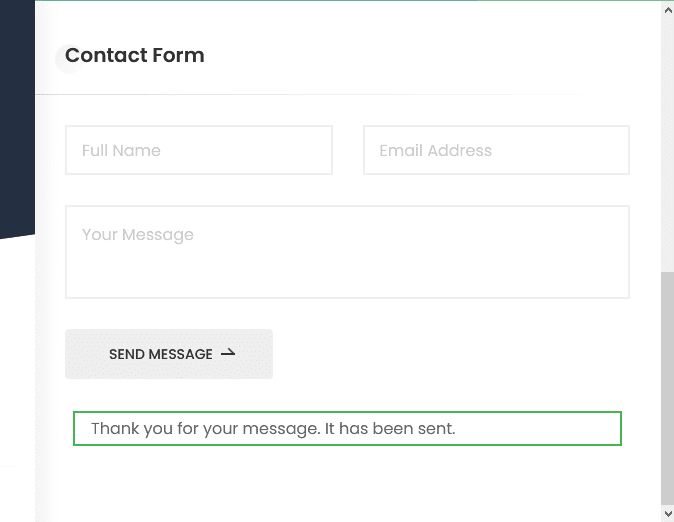A screenshot of a contact form is presented on a white background, framed by a thin green border along the top edge. Notably, a black strip with a diagonal edge runs halfway down from the top left corner to the center of the left side. The header, positioned at the upper left corner, reads "Contact Form" in bold black font, underscored by a thin gray line.

Beneath this header, three input fields are highlighted in a very light gray color: at the top left is "Full Name," to its right is "Email Address," and below these is "Your Message." All fields are currently empty. Below the message box sits a gray button with "SEND MESSAGE" written in black capital letters, accompanied by a half-arrow icon.

Under this button, outlined with a thin green line, is a notification box displaying the message, "Thank you for your message. It has been sent."

On the right-hand side of the image, scroll arrows are visible at both the top and bottom, with a gray vertical scroll bar situated in the bottom right-hand quadrant.